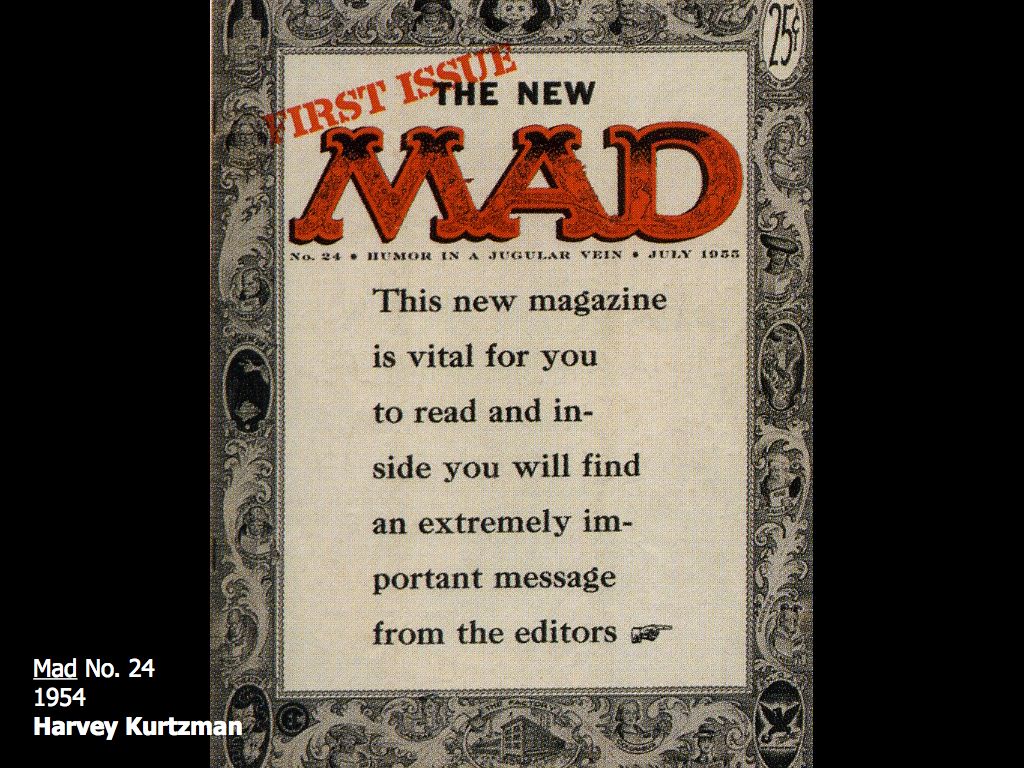This image is an intricately designed magazine cover, specifically the first issue of MAD Magazine. The cover flaunts an elaborate, presidential-themed border adorned with flourishes, eagles, and possibly images of presidents, setting a regal tone. Centered at the top of the cover is the iconic MAD character, Alfred E. Neuman, with his quirky grin. Below him, in bold red text, is the title "The New MAD," signaling its inaugural issue. Top left corner of the cover, the bold red text proclaims "First Issue." Directly beneath the title, the text reads, "Number 24: Humor in a Jugular Vein, July 1955." An eye-catching message urges readers, "This new magazine is vital for you to read and inside you will find an extremely important message from the editors," accompanied by a hand pointing to the right. The bottom left corner of the image, superimposed, declares in white text, "MAD Number 24, 1954 Harvey Kurtzman." The magazine's price, twenty-five cents, appears on the upper right corner. Despite references to being the first issue, the cover paradoxically marks it as number 24, contributing to the whimsical and perplexing nature of MAD Magazine.